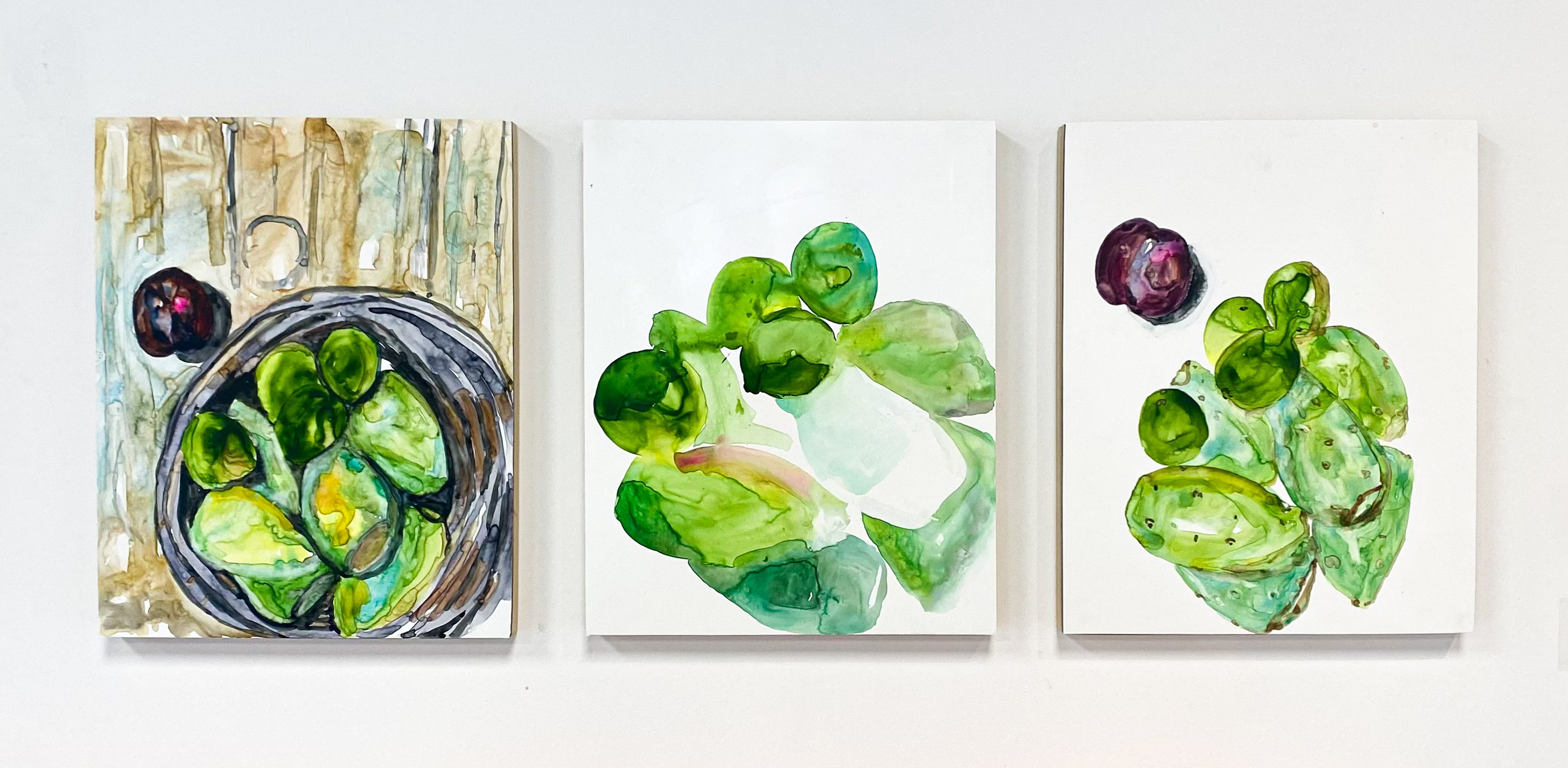The image is a cohesive triptych of three distinct but thematically connected paintings. Each painting is slightly oblong in a rectangular shape and hung side-by-side. The first painting on the left depicts a bowl filled with green fruit, possibly avocados or mangoes, placed on a wooden table, discernible by its striped texture. In the upper left corner of this painting, there is an ambiguous black and red item, difficult to identify. The central painting features an abstract arrangement of green items in a loose circular form set against a stark white background. This painting predominantly showcases various hues of green with a subtle streak of burnt orange. The rightmost painting mirrors the first with a circular grouping of green items, again likely avocados or mangoes, against a white backdrop. It also contains an indistinct red item in the upper left corner, further connecting the series through recurring elements and colors. Together, these paintings create a unified theme through their portrayal of green fruits, abstract shapes, and complementary color highlights.